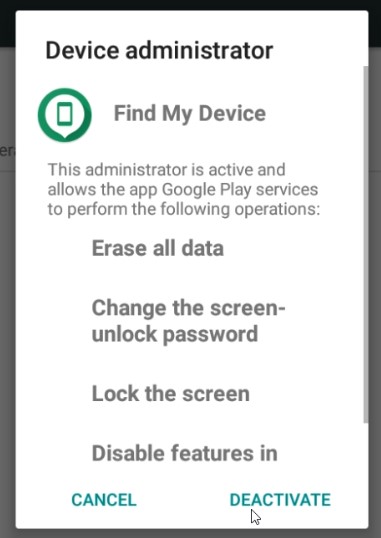The image depicts a website pop-up page, overlaying a web page with a top black banner and an underlying gray background that conceals the content behind it. The pop-up itself is predominantly white and stretches almost from the left to the right edge, with a slight margin of the background banner visible on either side.

At the very top of the pop-up, the title "Device Administrator" is prominently displayed in black text. Below this, there is a green circle with a smaller white circle contained within a green outline, followed by the text "Find My Device" in black on the right.

The information provided below explains that the "Device Administrator" is active and grants the Google Play services app permission to execute specific operations. The list of these operations is written in dark gray text and includes:
- Erase all data (in bold),
- Change the screen unlock password,
- Lock the screen,
- Disable features.

At the bottom of the pop-up, on the left side in green text, the word "Cancel" appears, while to the right, also in green, the word "Deactivate" is displayed, accompanied by a small white arrow pointing towards "Deactivate" below it. A gray scroll bar on the right-hand side indicates that more content is available below the visible portion of the pop-up.